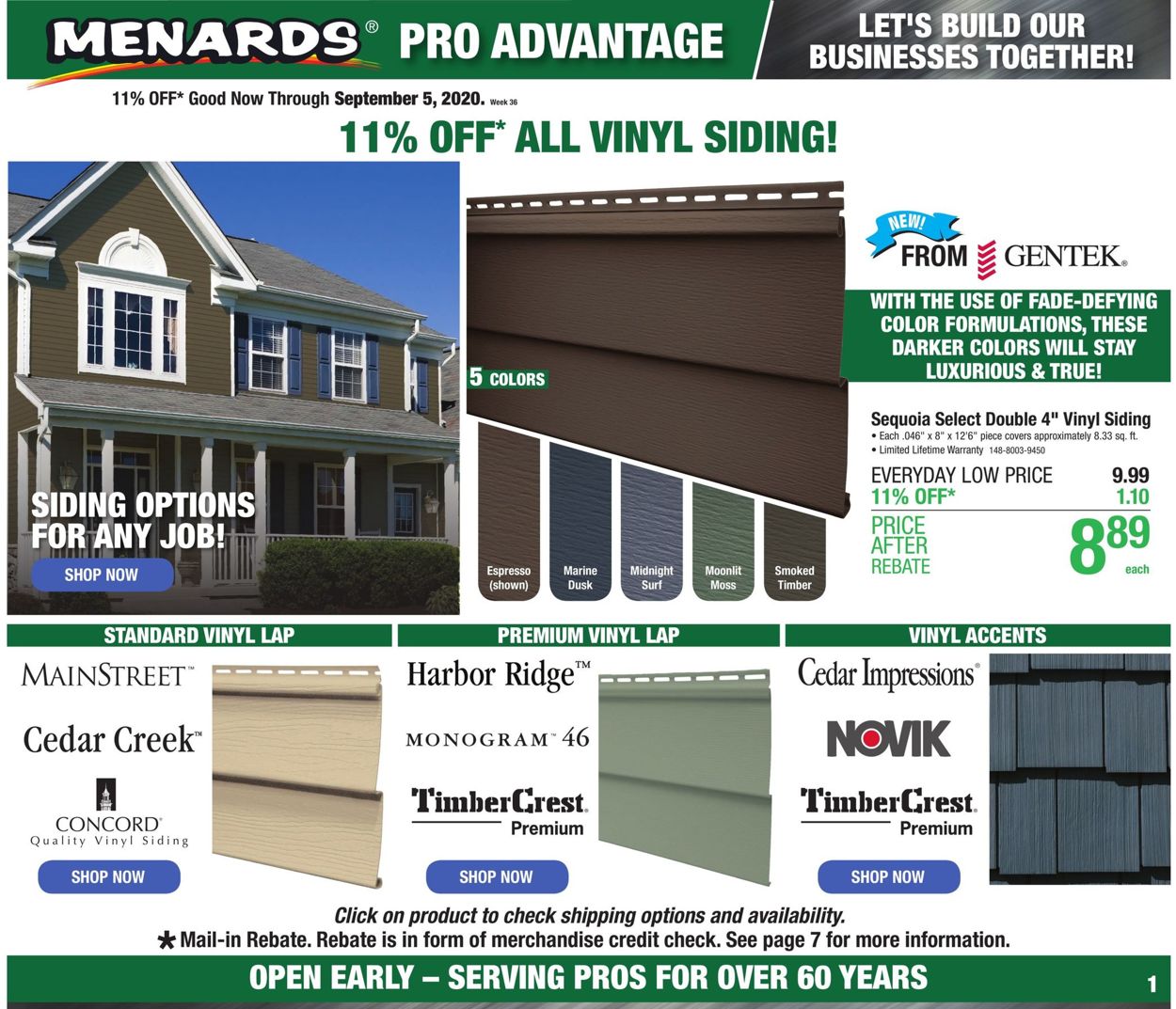**Menards Pro-Advance Promotional Image:**

This promotional image from the Menards Pro-Advance website features an appealing advertisement with the tagline, "Let's Build Our Business Together." Highlighted prominently is an 11% off promotion on all vinyl siding, valid through September 5th, 2020. 

The focal point of the graphic is an image of a house showcasing various siding options suitable for any job, complemented by the "Shop Now" button in blue. 

Central to the image is a display of five color options, with swatches hanging down, each clearly labeled to showcase the range of choices. Below this, there is a detailed section promoting the 'Sequoia Select Double 4-Inch Vinyl Siding' from Gen Tech. This section emphasizes the use of fade-defying color formulations ensuring that the darker colors remain luxurious and true. The product is listed with an everyday low price of $9.99, with the 11% discount reducing the final price to $8.89 after a rebate of $1.10.

Underneath this main promotion, there are additional images and descriptions for various other siding collections:
- Main Street
- Cedar Creek
- Concord (Shop Now button in blue)
- Premium options including Harbor Ridge, Monogram Timber Crafts (all with "Shop Now" buttons in blue)

Further, there's a dedicated section for Vinyl Accents showcasing Cedar Impressions, Novak, and Timber Crest Premium with "Shop Now" buttons.

At the bottom of the image, a green bar emphasizes Menards’ commitment with the statement "Open Early, Serving Pros for Over 60 Years." The image also mentions that the 11% rebate comes in the form of a merchandise credit check.